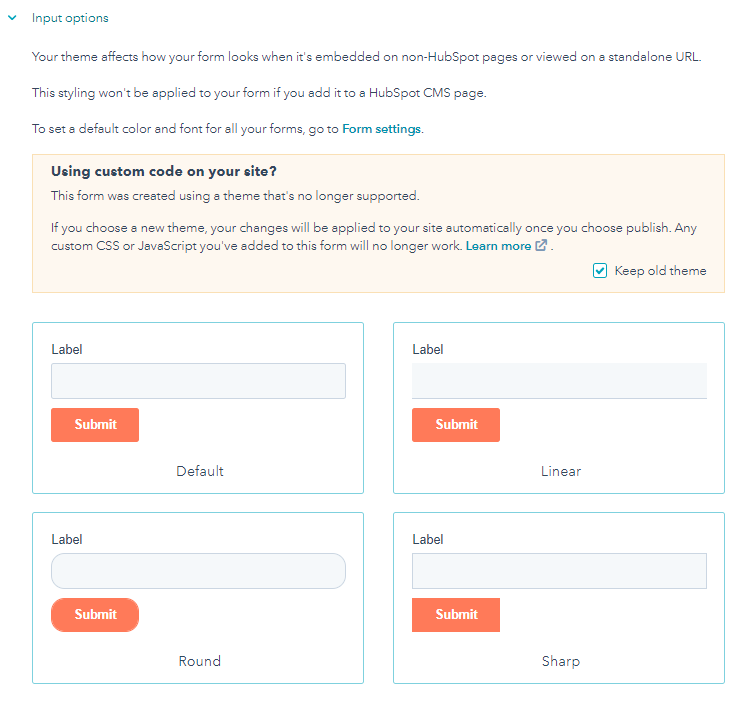This image features a screenshot of an online form customization interface. It displays a notice regarding "Input Options," informing the user that the theme affects how the form appears when embedded on non-HubSpot pages or viewed via a standalone URL. A note clarifies that this styling won't apply if the form is added to a HubSpot CMS page and directs users to form settings to set default color and font for all forms. Additionally, it mentions that using custom code on the site, the form was created with a theme that is no longer supported. Users are advised that selecting a new theme will automatically apply any changes upon publishing, but any custom CSS or JavaScript previously added to the form will cease to function. 

In the bottom right corner, there is a "Learn More" button adjacent to a checked checkbox labeled "Keep old theme." The interface also includes four text boxes with corresponding labels: the upper left text box is labeled "Label," with a "Submit" button beneath it. The remaining three text boxes have unique labels positioned in their bottom centers: "Default" for the bottom center box, "Linear" for the upper right box, "Round" for the bottom left box, and "Sharp" for the bottom right box.